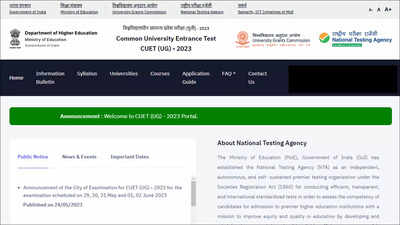This screenshot, captured from a computer, is a horizontal rectangular image displaying text that is notably blurry. At the top left of a white section, the discernible black text reads "Department of Higher Education." To its immediate right, the text states "Common University Entrance Test 2023." Beneath this, a horizontal blue bar spans the width of the image, containing white text that includes clickable options such as "Home," "FAQs," and "Contact Us." Below the blue bar, a green bar with white text is visible, though the specific wording is unclear apart from fragments like "Welcome to" and "2023." The lower portion of the image features a white section with black text. On the upper left side of this section, a blue underlined word appears, though it remains indistinguishable. Dominating the right side of this white field, a text heading reads "About National Testing Agency," leading into a comprehensive paragraph beneath it.